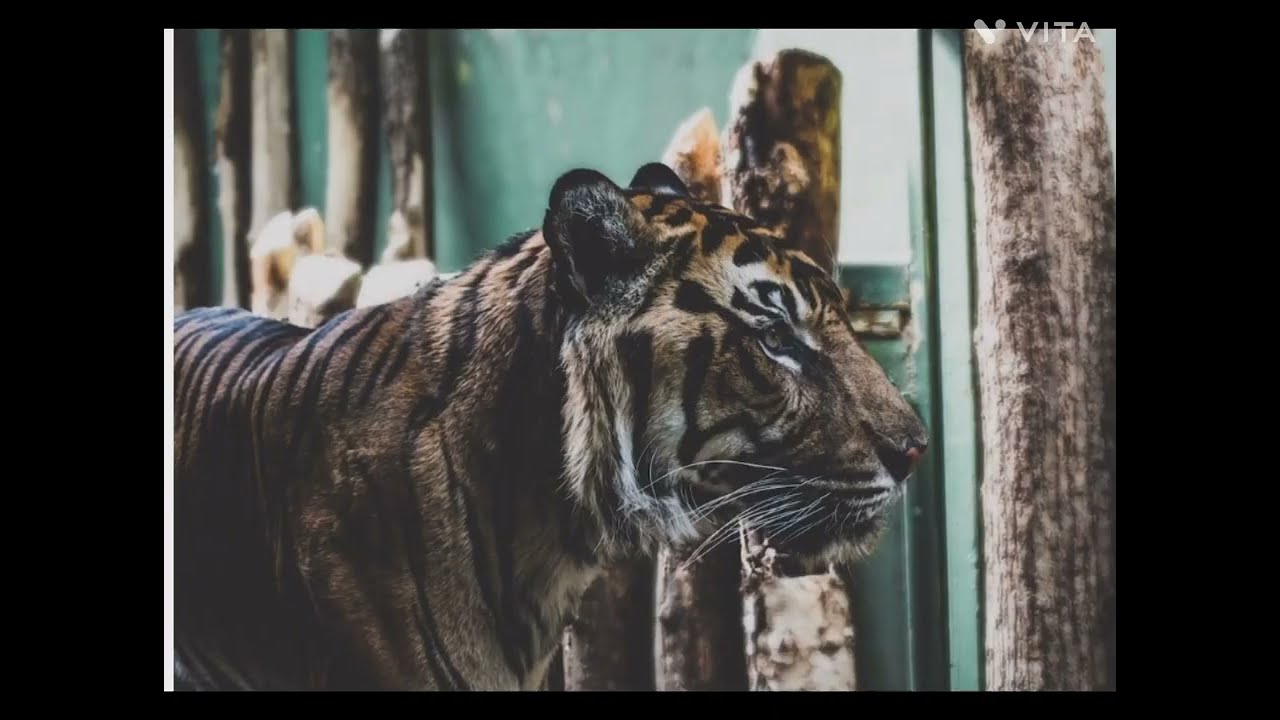This detailed photograph captures a majestic tiger, predominantly dark in color, leaning more towards brown with black stripes than the typical orange. The side view showcases the tiger's intense look as it gazes to the right, possibly outside of a cage. The white markings above its eyes and around its neck suggest an older tiger, adding to its distinguished appearance. The focal point of the image, the tiger occupies the center and commands attention, especially with its head positioned directly at the middle. In the background, a jade green wall and a man-made wood fence emphasize a zoo setting. The image features muted tones of green, brown, black, gray, and a hint of red. Completing the scene is a logo "VITA" in the upper right corner of the photograph, which appears to be extracted from a video frame.